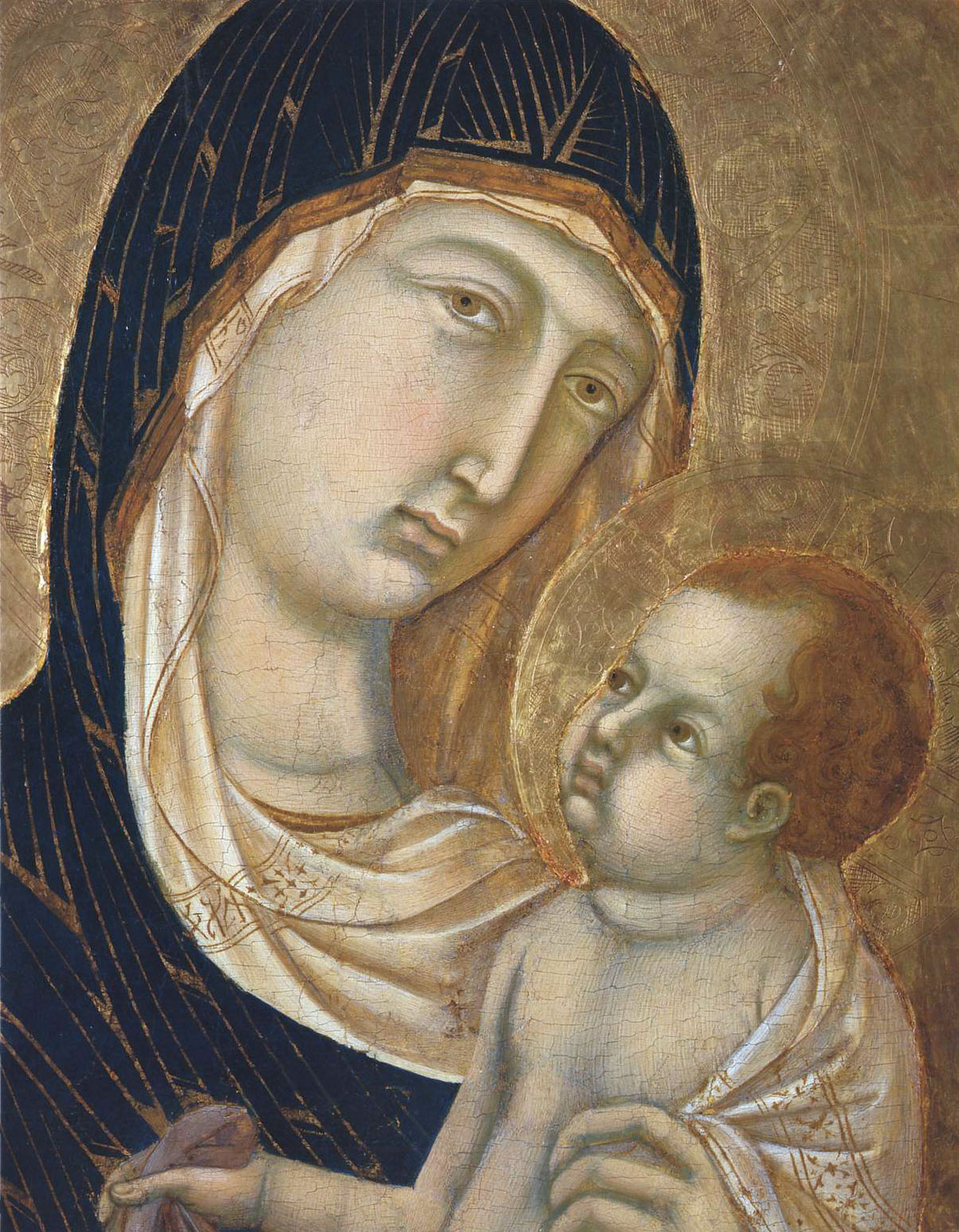The painting, likely from the Italian Renaissance period, depicts the Virgin Mary holding baby Jesus. The Virgin Mary is dressed in a blue cloak adorned with gold markings, draped over her head and shoulders, covering a white veil beneath. Only her face and a little past her shoulders are visible. She is looking down at baby Jesus with a tender expression. Baby Jesus, portrayed with rust-colored hair, is dressed in white and is clasping part of the Virgin Mary's cloak with his left hand. His figure is shown from the waist up, and he gazes up at his mother longingly. The background of the painting is an abstract brownish beige, giving the scene an almost ethereal quality. The mother is positioned on the left and the child on the right, creating a harmonious composition typical of traditional religious iconography seen in many churches.